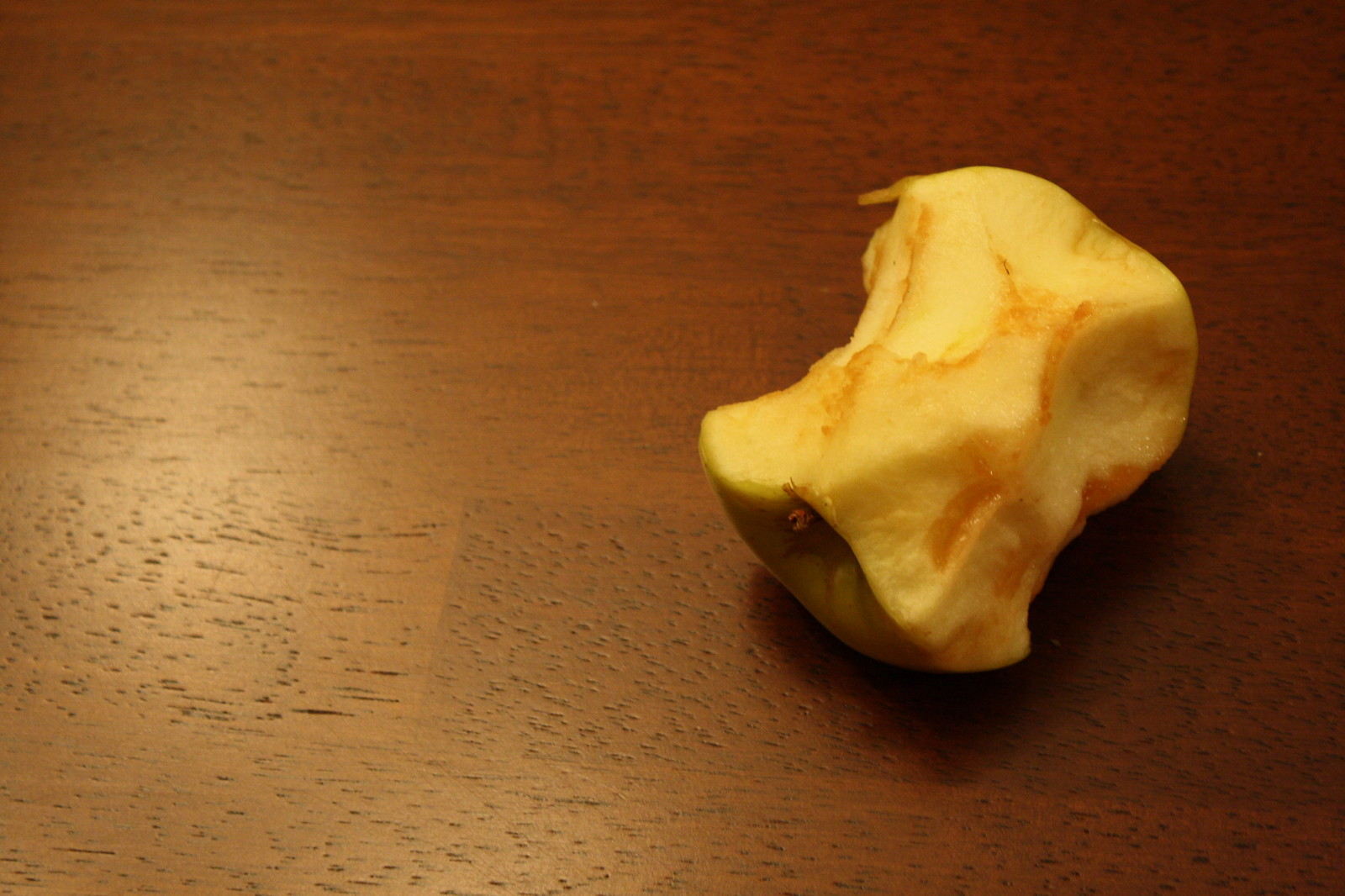The image features a close-up view of a half-eaten green apple, which has been left to rot on a wooden tabletop. The apple, with its green skin still visible on the left side, shows extensive signs of aging and decay, including brown discoloration around the bite marks. The rotting flesh, characterized by pronounced brown lines, indicates that the apple has been decomposing for quite some time. A small portion of the stem remains attached, protruding from the top. The background showcases a dark cherry wood table with visible indentations and pits, highlighted by a glare on the left side, suggesting the authenticity and ruggedness of the wooden surface. The primary focus of the image is this deteriorating apple, which is evidently no longer fit for consumption and should be disposed of immediately to prevent further decay.